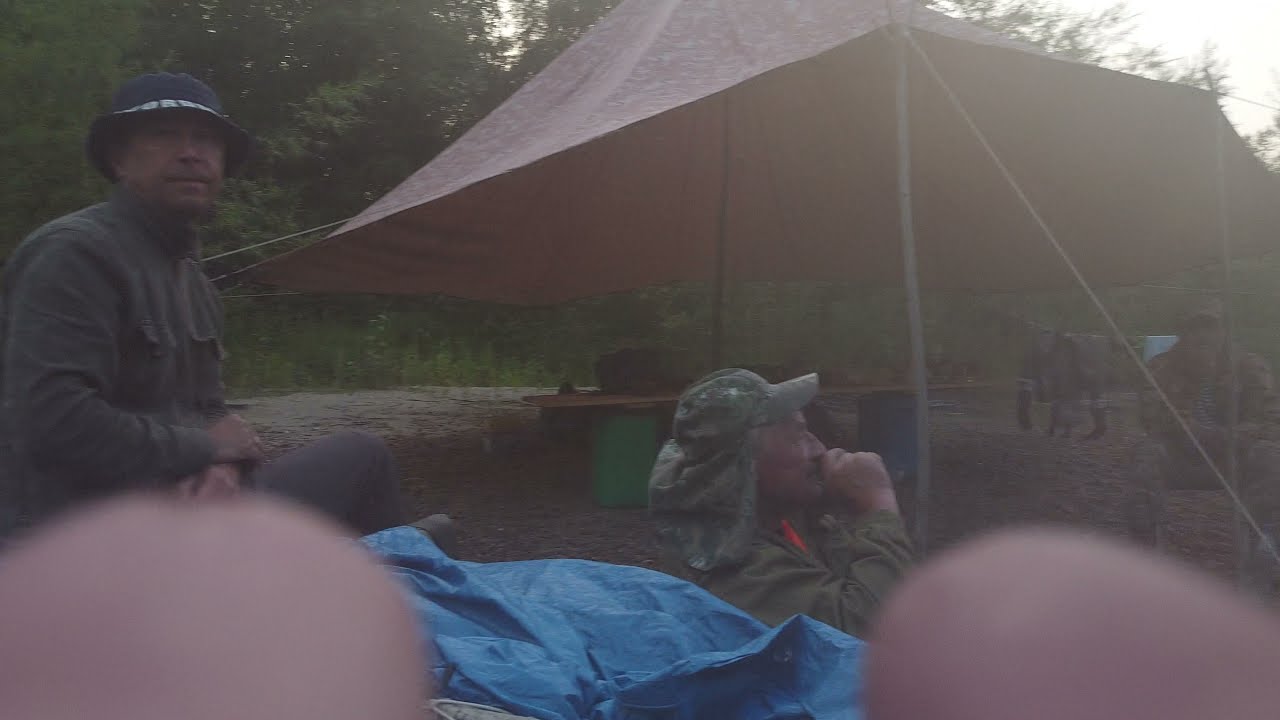This exterior daytime photograph captures a group of men in what appears to be a forest setting, shrouded by a thick whitish-gray haze. A large brown tent, mounted on wooden sticks and secured with ropes, dominates the center of the scene. The tent, which serves as a canopy, is made from a brown tarp and shades a makeshift wooden table supported by blue and green cases. 

To the left of the tent, a man with brown skin wearing a floppy black hat and a dark green long-sleeved shirt sits cross-legged, looking towards the camera. His arms are crossed in front of him. Adjacent to him in the middle of the image, another elderly man with brown skin is seen in a sitting position. He is wearing a moss green cap with a neck shield and a matching long-sleeved shirt. He has an orange detail on his shirt and has his hand up to his mouth, facing towards the right in profile. Further to his right, another individual clad in mottled green clothing and cap is partially visible, seated and facing the camera.

The bottom of the photograph is partially obscured by two large tan-colored blobs, likely the fingers of the person taking the picture, with a crumpled blue tarp situated between them. In the backdrop, the forest is dense with trees and a grass-filled ground. There are also clothes hanging on a line, adding to the rustic, makeshift atmosphere of the campsite.